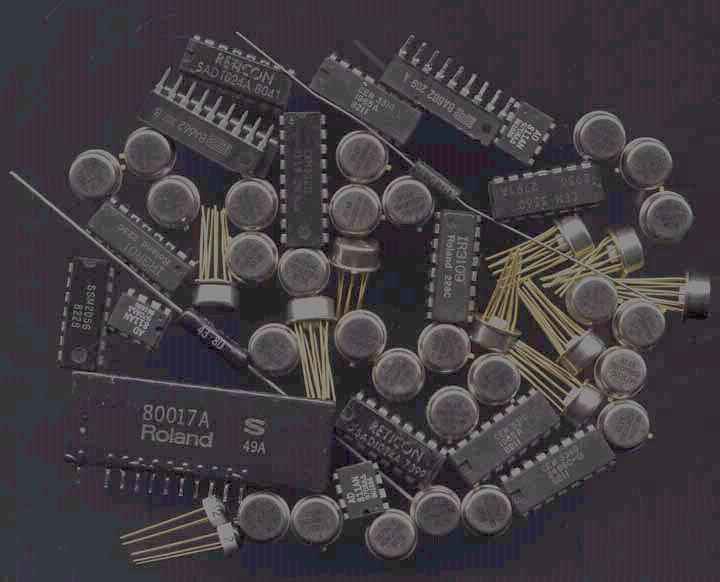This rectangular image offers a bird's-eye view of a cluttered surface, possibly a workbench or countertop, featuring a pixelized purple and green background. Scattered across this space are various tools and components, predominantly drill bits arranged in multiple rectangular holders. These holders contain an assortment of drill bits of different sizes, each marked with various labels and numbers, such as "80017A Roland" and "S490A." Among the items are several small, round, silver caps, some oriented upwards, while others lie on their side. These caps appear to have thin, toothpick-like extensions, possibly wires, protruding from them, giving them a cap-like appearance. The rest of the items seem to be electronic components, including transistors and other metal parts, some dark and others light. The overall scene appears disorganized, with no distinct pattern to the arrangement of these varied objects.